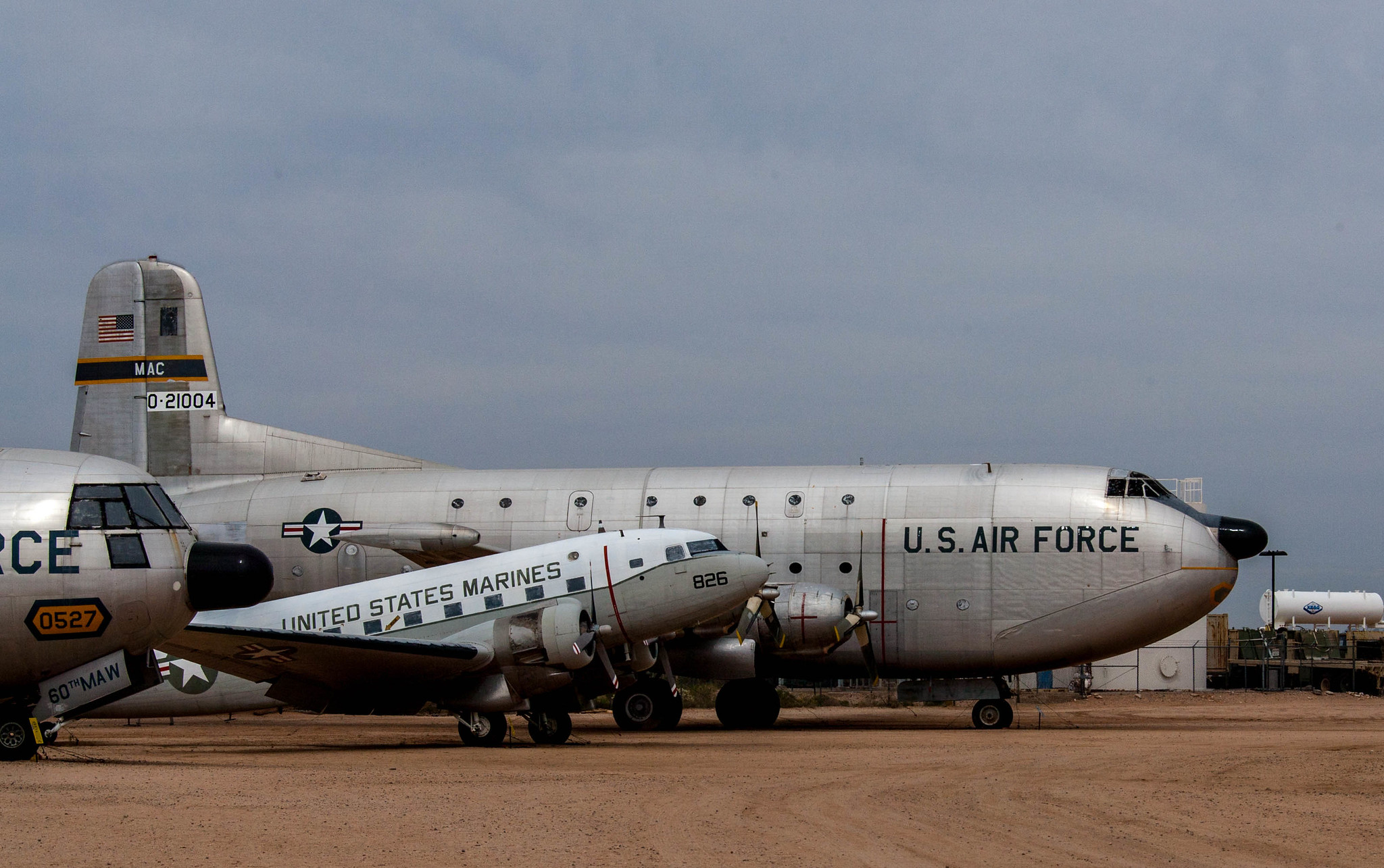This outdoor photograph at a military base showcases three older military aircraft with likely propeller designs. Dominating the background is a large gray plane marked with "U.S. Air Force" and a distinctive star insignia, along with "MAC" in white letters on a blue stripe, and the serial number "021004" on the tail. To the side and slightly in front of this aircraft is a smaller white and gray plane labeled "United States Marines," featuring the number "826" near its nose. The closest plane's front end is partially visible, displaying an orange marking with the numbers "0527." The scene unfolds on a brown tarmac, marred with tire tracks, possibly hinting at a Vietnam War-era base. A white fuel tank and a partly cloudy blue sky form the backdrop for this detailed military scene.